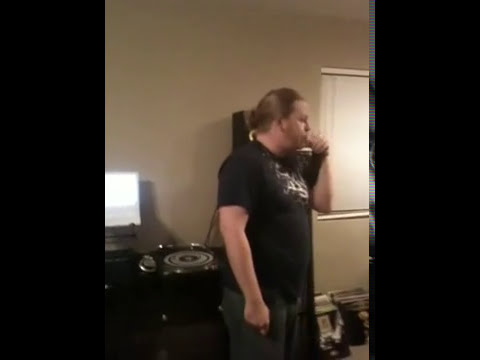The image features a young man with light brown hair pulled back into a small bun or ponytail. He is wearing a black t-shirt with a white design on the front and gray sweatpants. The man appears to be drinking a shot of alcohol, holding a small shot glass to his lips and tilting it back. He is standing in a room that looks like a living room or an office within a house that seems dedicated to playing records. 

The room has off-white or beige walls and minimal view of a light-colored floor. Positioned in the center of the image, the man is seen from a side view, facing right. Behind him and slightly to the left are blinds covering a window. To his immediate left (facing the image head-on) is a black and gray record player sitting on a black table. Adjacent to the table on the left is a lamp, casting a white light. In the bottom right of the image, two rows of vinyl records can be spotted on the floor. The overall scene is captured with a somewhat blurry quality, adding a sense of casual, everyday atmosphere to the setting.